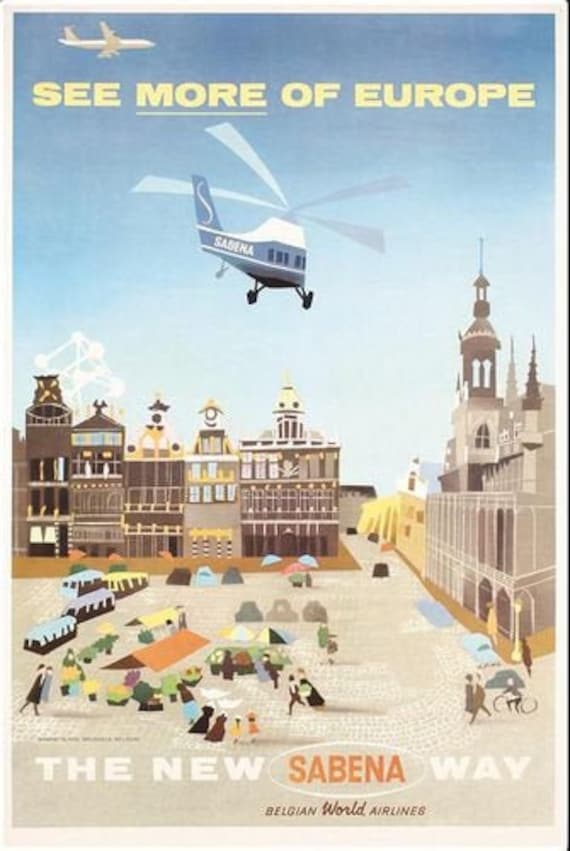This image features a detailed and colorful poster promoting Belgian World Airlines, with vibrant illustrations encompassing various elements of a lively European scene. At the top, the bold and eye-catching text "SEE MORE OF EUROPE" is written in large, capital, yellow letters against the blue sky. Below this, a white airplane is seen flying towards the right, while a helicopter with a blue and white fuselage and light blue propellers hovers beneath it. The helicopter also has blue tail wings and black wheels clearly visible.

Dominating the middle section of the poster are detailed depictions of various buildings. On the left side, there are brown and beige buildings adorned with gold trim and white tops, interspersed with a distinctive Ferris wheel in the back left corner. To the right, several buildings of brown and yellow hues are shown receding into the distance, with a prominent gray building featuring brown detailing closer to the foreground.

The ground is depicted as light brown and cobbled, bustling with activity. There are numerous tents in vivid colors such as orange, yellow, green, and blue. Among these are small housing areas painted in shades of gray, as well as light blue umbrellas scattered throughout. People in brown, gray, black, and blue clothing walk amongst the scene, interspersed with blue, yellow, and brown buses and cars. At the bottom of the poster, the text "THE NEW SABINA WAY" is highlighted in white with a dark brown background, accompanied by the phrase "Belgian World Airlines" beneath it.